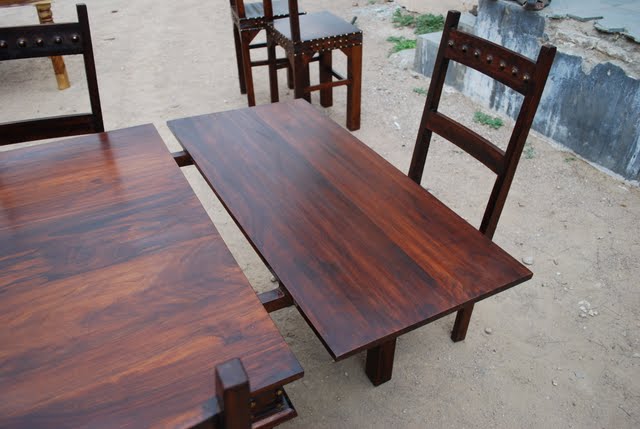The image captures a beautifully finished wooden table, seemingly outdoors on a dusty, light brown dirt surface. The table, a blend of rich dark wood with streaks of red reminiscent of cherry or mahogany, features an extended leaf, displaying its frame underneath. The wood grain of the table surfaces shows unique directions, suggesting an additional leaf has been added at the end. Surrounding the table are four simple, dark wooden chairs, their tops adorned with circular designs and the seats possibly featuring detailed patterns. The chairs are grouped around the table, positioned on an off-white or dusty floor, while the backdrop reveals a rough, crumbling structure, likely concrete, adding a rustic charm to the scene.